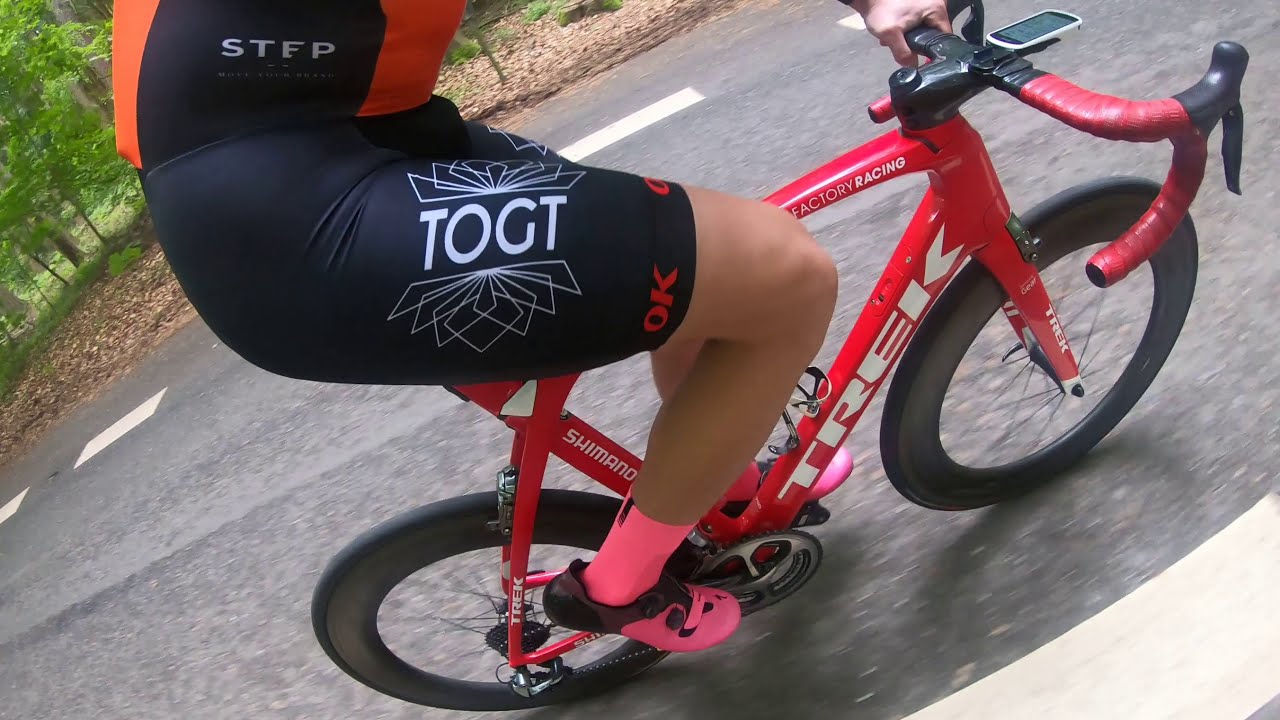The image is a horizontally aligned rectangular photograph taken outdoors, depicting the lower half of a cyclist in motion against a bright and clear backdrop. The cyclist is riding a red 10-speed style bike with the words "Shimano Trek" and "Factory Racing" inscribed on the frame. The bike features curved handlebars wrapped in red tape with black brakes, and black wheels. The rider is seen wearing black biker shorts with white "T-O-G-T" lettering and red "OK" at the hem. The tight-fitted top is black on the sides and orange on the front and back, with the letters "S-T-F-P" visible on the side. The cyclist's attire includes vibrant pink socks and matching pink shoes with black accents.

The setting is a street marked by white dashed lines, indicating a lane, with a background of lush green trees and brown elements on the ground that could be dead leaves or mulch. The image captures the motion of the cyclist, with slight streakiness at the bottom suggesting movement, and is taken during daylight, ensuring plenty of natural light. No other cyclists are present in the scene.